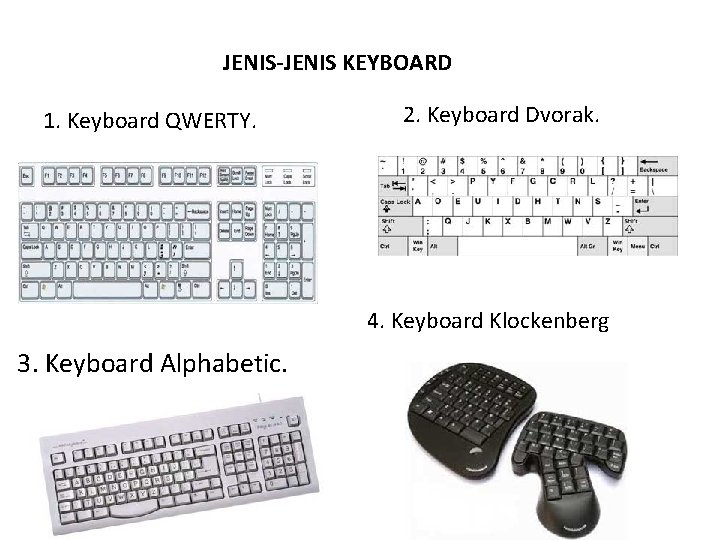This image, which appears to be an advertisement, features different types of keyboards against a plain white backdrop. At the top in bold black text, it reads "Genus-Genus Keyboard." The image is sectioned into four labeled parts:

1. **Keyboard QWERTY** - Shown in the top left, this is a standard QWERTY keyboard. The keys are white, with gray secondary keys, including the function keys (F keys) at the top.

2. **Keyboard DVORAK** - Positioned to the right of the QWERTY keyboard, this one is labeled number 2. It’s a more simplified, narrow keyboard without function keys, and it features a unique key arrangement differing from the standard QWERTY layout.

3. **Keyboard Alphabetic** - Located in the bottom left and labeled number 3, this keyboard arranges keys alphabetically (ABCDE format) instead of the traditional QWERTY layout. It has a number pad on the right, giving it a more retro or old-school appearance.

4. **Keyboard Klokenberg** - Featured in the bottom section labeled number 4, this is a distinctive ergonomic, two-piece keyboard. Both pieces are black, designed to provide a more comfortable typing experience by allowing each half of the keyboard to be positioned to better suit the user’s hand placement.

Overall, the image exhibits diverse keyboard layouts, showcasing variations from traditional to ergonomic designs.